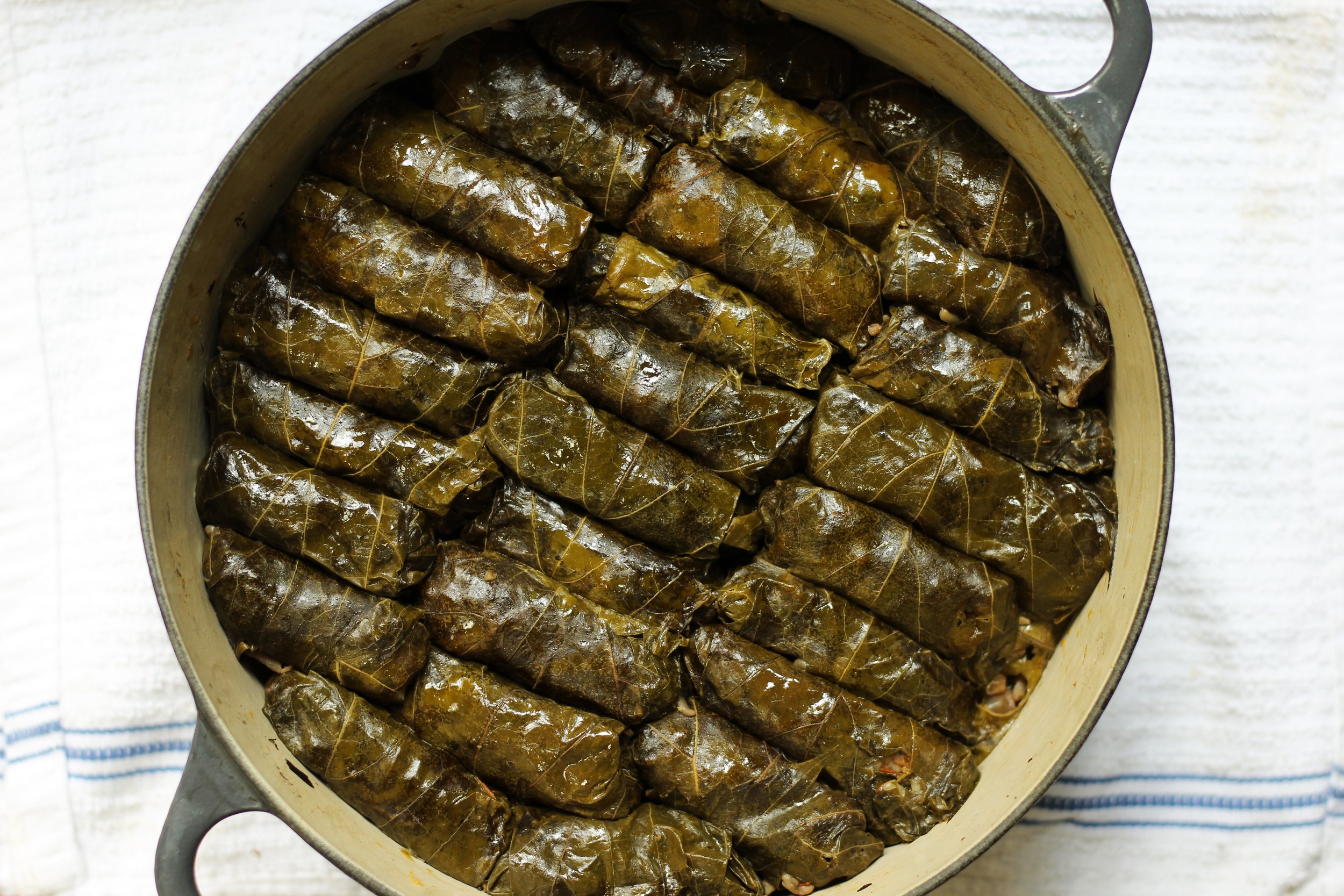A bird's eye view photograph showcases a large cooking pot, steel or cool gray in color, complete with two handles, partially visible. Nestled within the light tan interior of the pot are several neatly arranged rolls, wrapped in what appears to be seaweed or some type of leafy plant. The pot rests on a kitchen towel, distinguished by its fabric texture and a single blue stripe running horizontally across the bottom, invoking a classic kitchen aesthetic.